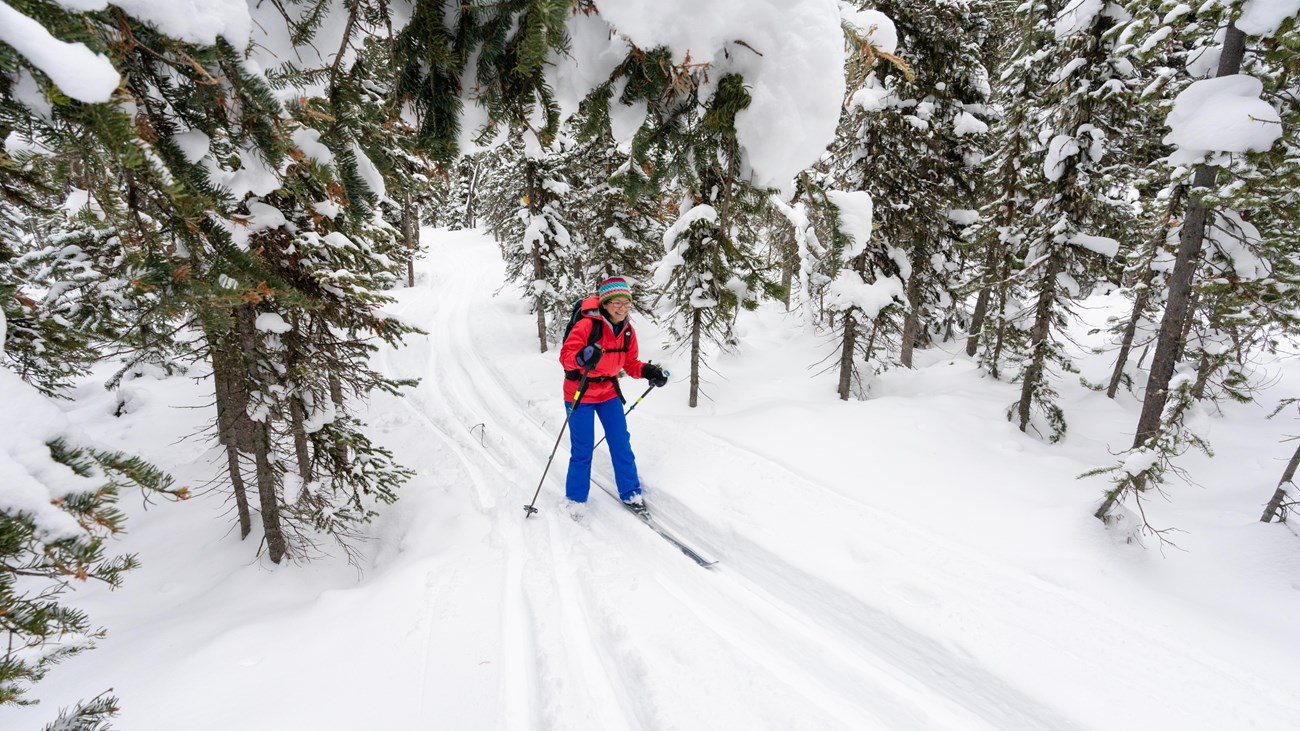The image depicts a female skier in a snowy, forested landscape, framed by tall, snow-covered pine trees. She stands upright, moving at a leisurely pace along well-worn ski tracks in fairly deep, white snow. The surrounding trees are laden with heavy clumps of snow, casting slight shadows that darken the snow around their bases. She is dressed in vivid blue ski pants, a bright red winter ski jacket, black gloves, and a knit beanie. An orange backpack, which matches the beanie, is visible due to some straps and a bulge in the background. The skier’s fair skin is discernible, and she exudes an eager expression as she holds her ski poles. The daylight scene, possibly on a cloudy day, provides even lighting that illuminates the skier and the pristine winter environment.